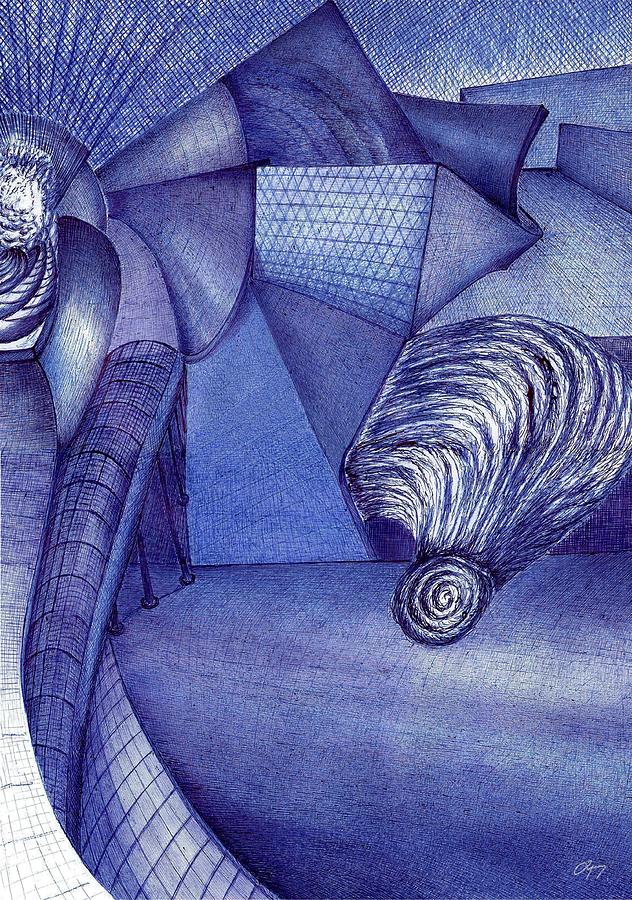This abstract artwork is a poster-sized print set against a predominantly blue background, resembling a blue jean material in certain spots, and an ink pen texture in others. The top of the image features an intricate network of lines and geometric shapes, including an array of triangles and bent triangles pointed to the right, as well as what appears to be a mesh ceiling formed from numerous X’s. These elements contribute to a textured canvas surface, especially visible at the top left and right corners.

Descending from this structured top, the artwork contains various geometric forms, including squares, square-type patterns, and cone shapes that seem almost cushion-like, perhaps forming a distorted couch. The central focus is a complex coil composed of numerous fibers in shades of black, white, and blue, creating a spiral ball. This coil rests on a cushion-like surface that appears solid blue with an iridescent quality and is intersected by a darker, criss-cross arm pattern. 

The lower sections of the image present a grid drawing on the lower left, transitioning upward into clusters of smaller squares and adjacent triangles, all predominantly blue. Waves, primarily white with hints of blue, occupy the upper left corner, intersected by ascending dark blue lines. Overall, the background maintains a grid-like pattern, harmonizing the intricate abstract details with a mix of white, dark blue, and sporadic touches of black, completing this dynamic and textured composition.